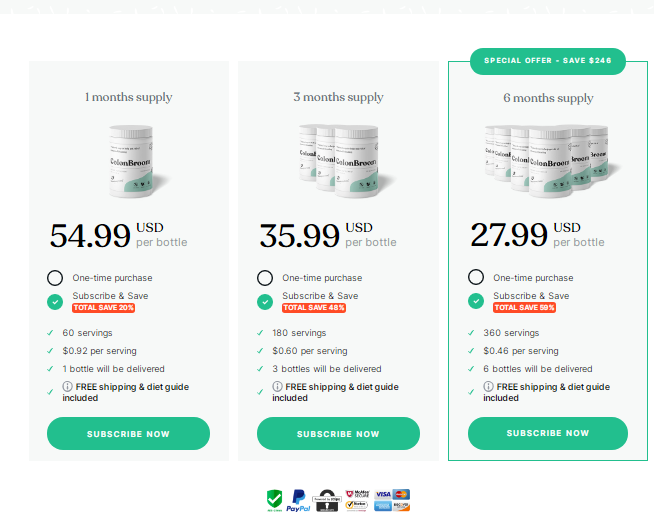The image displays three vertically aligned, lightly shaded gray rectangles, with each representing different subscription plans for "Colon Broom" pill bottles. 

**Left Rectangle - One Month Supply:**
- At the top, in small dark gray font, it reads "One Month Supply."
- Below, a pill bottle labeled "Colon Broom" with a white body and a light mint accent at the bottom right is depicted.
- In large black font, it lists the price as "$54.99 USD per bottle."
- Below the price, the options "One Time Purchase" or "Subscribe and Save" are available. The "Subscribe and Save" option is selected, indicated by a greenish circle to the left.
- An orange box beneath this selection notes a total savings of 20%.
- Further details include "60 servings," costing "$0.92 per serving," with free shipping and a diet guide included. It prompts users with "Subscribe Now."

**Middle Rectangle - Three Month Supply:**
- Titled "Three Month Supply."
- Features three pill bottles arranged diagonally from left to right.
- Lists the price as "$35.99 USD per bottle."
- Offers the same subscription options: "One Time Purchase" or "Subscribe and Save," highlighting a total savings of 48%.
- Specifies "180 servings" at "$0.60 per serving."
- States that three bottles will be delivered and encourages to "Subscribe Now."

**Right Rectangle - Six Month Supply:**
- Labeled "Six Month Supply."
- Displays six pill bottles.
- Shows the price as "$27.99 USD per bottle."
- Provides "One Time Purchase" and "Subscribe and Save" options, with a highlighted savings of 59%.
- Details "360 servings" at "$0.46 per serving."
- Mentions that six bottles will be delivered and includes a prompt to "Subscribe Now."